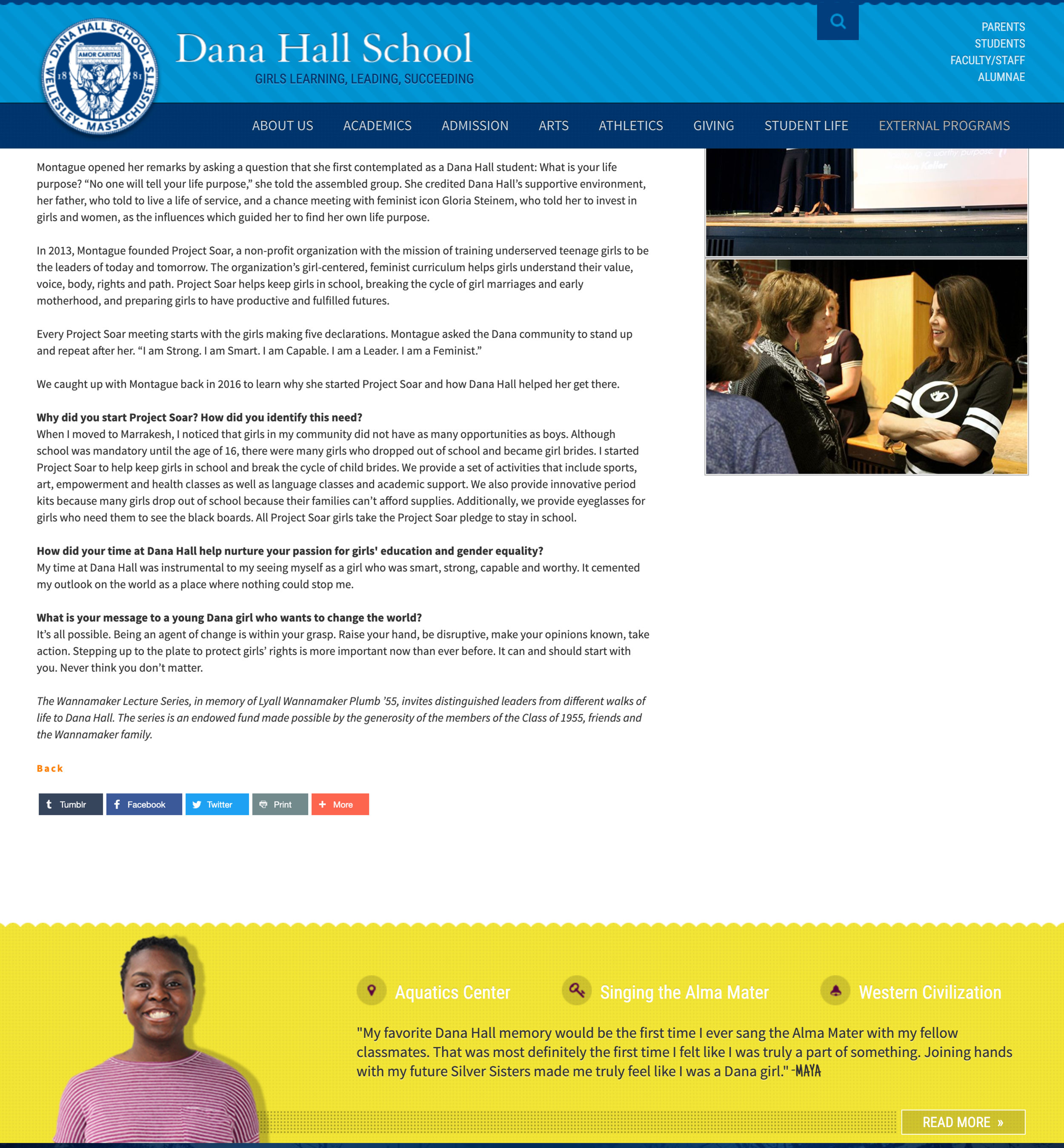The image features a white background with a light blue border surrounding the content. At the top, "Dana Hall School" is prominently displayed. Below it, there is a blue square containing a blue, medium-toned magnifying glass. Adjacent to this square are several blue rectangles, each labeled with different categories: "About Us," "Academics," "Admission," "Arts," "Athletics," "Student Life," and "External Programs." Notably, the "External Programs" label is in beige. 

Beneath these categories, there is some additional information. At the bottom of this section is an orange button labeled "Back."

Toward the center of the image, there are two photographs. The first photograph appears to depict an assembly with someone speaking on stage. The second photograph seems to capture a moment after the assembly, featuring a few women engaged in conversation.

At the lower part of the image, a yellow rectangle contains the image of a smiling woman. Accompanying this image are the phrases: "Aquatic Center," "Signing the Alma Mater," "Western Civilization," and "My favorite Dana Hall memory would be the first time I ever sang the Alma Mater with my fellow classmates."

To the bottom right, there is a light brown rectangle with the words "Read More," providing an option for additional information.